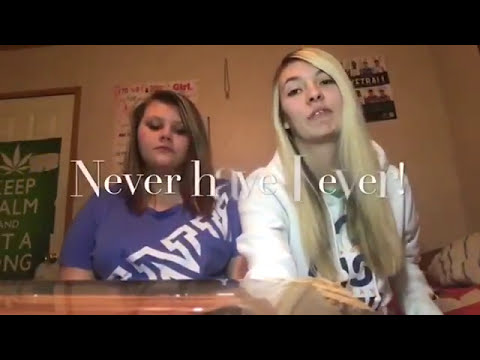Two young women are sitting side by side at a table, seemingly recording a video for YouTube or Facebook, as suggested by the caption in the middle that reads, "Never Have I Ever." The one on the right is wearing a purple shirt with white lettering, while the one on the left, donning a white shirt with gray and black lettering, has long blonde hair reaching down to her elbows with streaks of black near the roots. The woman in the purple shirt has shorter, brown hair extending just past her shoulders. They are situated in a room with tan walls, featuring posters behind them; one is green with a marijuana leaf and the words "Keep Calm," and another is white. The scene suggests they might be sitting on a bed, with a desk or shelf in front of them. The overall setting and their focus on the camera indicate that this image is a screenshot taken from a video, likely involving a game of "Never Have I Ever."